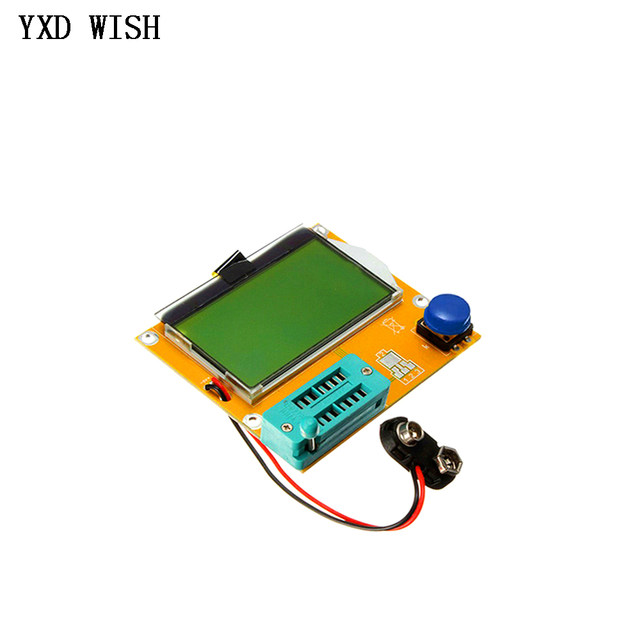This color photograph features an orange circuit board floating against a white background. In the upper left corner, black text in all caps reads "YXD WISH." The central focus of the image is the circuit board, which boasts several distinct components. The top half features a greenish touchscreen, possibly an LCD screen, covered with a piece of plastic. The lower left corner showcases an aqua-colored, screwed-on rectangular shape and the lower right corner contains a blue button. Extending from near the touchscreen are black and red wires ending in a black oval piece with two silver devices, likely for connecting a 9-volt battery. The circuit board is oriented such that this description matches its current angle in the image.